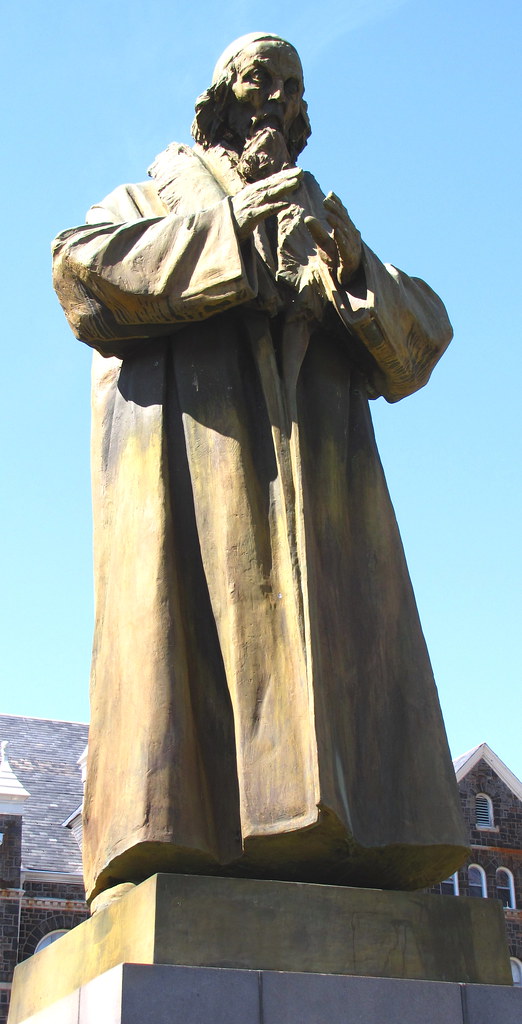The photograph captures a rough-hewn statue of a bearded man, adorned in a long robe with wide sleeves, and wearing a skullcap. His hands are in front of his chest, possibly in a gesture of prayer. The statue sits atop a rectangular, light brownish pedestal supported by a white stone base that disappears off the bottom of the image. The statue's material presents a textured palette of yellows and grays, highlighting its detailed craftsmanship. Our perspective looks up at the figure, allowing for a vast expanse of blue sky that transitions to a darker hue higher up in the frame. Flanking the statue are buildings on both sides; the structure on the right features gray and brown brick with white trim, while a similar building is visible on the left, set against the backdrop of the light blue sky.